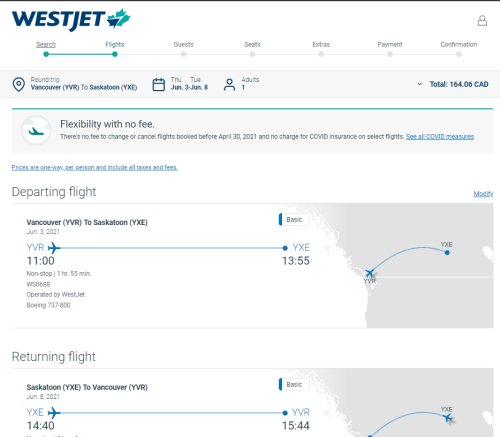Screenshot of a WestJet Airways Transaction Page: The image showcases a screenshot of the WestJet Airways website, prominently featuring their logo in the upper left-hand corner. The logo includes a Canadian maple leaf, underscoring that WestJet is a Canadian airline. The WestJet name is displayed in a bright, dark blue font, drawing immediate attention as the most prominent feature on the page. 

Below the logo, the itinerary search criteria are displayed, revealing a planned trip from Vancouver to Saskatoon. The travel dates specified are from June 3rd to June 8th, and the search is for a single ticket. This search bar is situated directly below the WestJet symbols, making it a key element of the page.

Beneath the search criteria, the results of the search are presented, detailing two specific flights—one for departure and one for return. The flights are described with all pertinent details, including departure and arrival times, duration, and the lack of stopovers. Despite being domestic flights within Canada, they account for sufficient duration and time zone changes. Additionally, two small maps provide visual representations of the flight paths, illustrating the direct routes and takeoff times without any layovers.